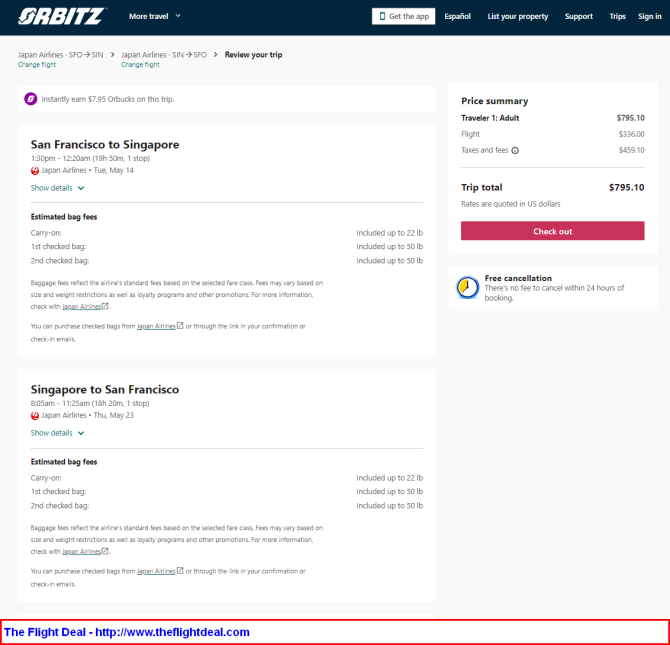This image is a detailed price quote for a car rental from Orbitz. The top of the page features a black rectangular banner with the Orbitz logo and the tagline "more travel" in white text. Adjacent to this banner, on the right side, there is a smaller white rectangular button labeled "Get the App." Additional categories are listed at the top, including an option to "List Your Property," though some text is unreadable.

As you scroll down, the main content area displays text in black on a white background. It indicates a trip from "San Francisco to Singapore." To the right, there is a "Price Summary" section for one adult traveler, showing a total amount of $7,951.10. Beneath this, the trip total is reiterated as $7,951.10. Directly below, a prominent red rectangular button with white text prompts users to "Check Out."

On the left side, there is a section titled "Estimated Bag Fees." Below this, the itinerary details "Singapore to San Francisco," along with specific departure times that are unclear. At the very bottom, a white rectangular box outlined in red features bright blue text advertising "The Flight Deal," including a URL link for further details.